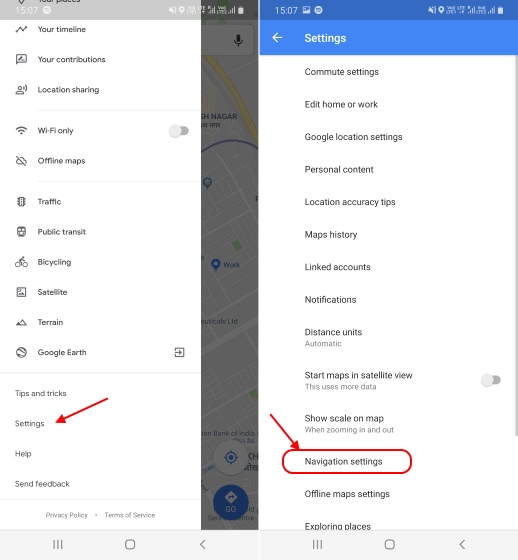This image consists of two separate screenshots taken from a mobile device displaying different sections of the Google Maps interface. The mobile toolbar at the top shows the time, Wi-Fi strength, cell service strength, and battery level, confirming it's a mobile device. 

The first screenshot features a partially visible map beneath a large menu covering most of the screen. This menu lists various options, each with its own icon: Your Timeline, Your Contributions, Location Sharing, Wi-Fi Only, Offline Maps, Traffic, Public Transit, Bicycling, Satellite, Terrain, and Google Earth. At the bottom of this list are additional options: Tips and Tricks, Settings, Help, and Send Feedback. A prominent red arrow has been added, directing attention towards the "Settings" option.

The second screenshot reveals the contents of the Settings menu, selected from the previous screen. Within this menu, different categories are displayed, including a section labeled "Navigation Settings," which is highlighted by a red circle. Another red arrow draws attention to this section, indicating that the user is providing step-by-step instructions, likely intended to guide someone through the settings process on Google Maps.